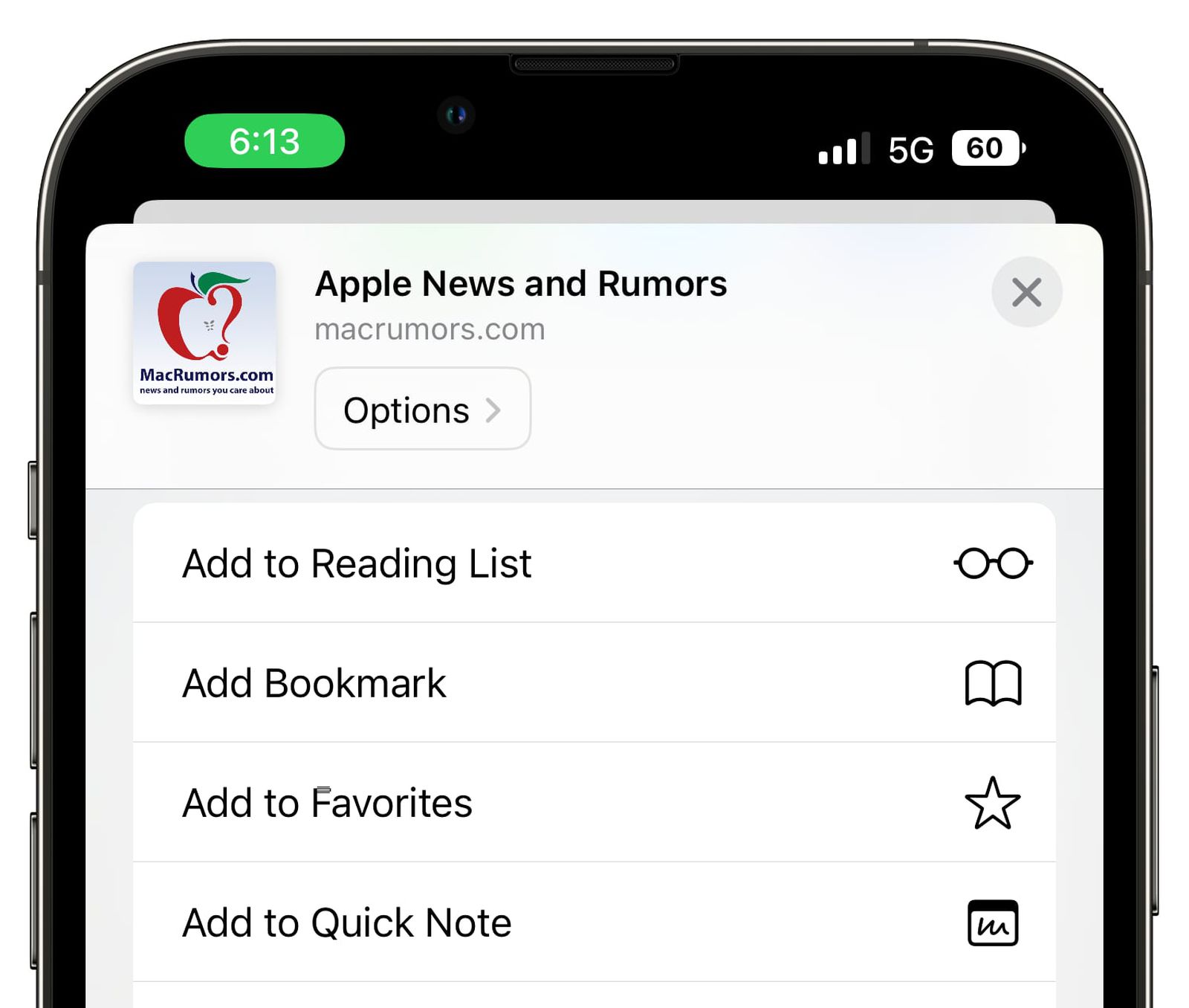A screenshot of a cell phone is displayed, showcasing a web page at the top of the screen. The phone's outline is highlighted in a green bubble, and the time reads 6:13. Subtle curved arrows form a circle at the top, accompanied by three out of four signal bars, indicating a 5G connection and a battery health of 60%.

The website in view is from MacRumors, prominently featuring the MacRumors logo—a white square with a cartoon-style apple where the right side forms a question mark, topped with a green leaf. The text beneath the logo reads "MacRumors: News and Rumors you care about."

On the far right of the screen, there is an 'X' symbol, which allows the user to close the page. Beside it is a bubble labeled "Options," containing a dropdown menu with four items: 
1. "Add to Reading List" with an icon of reading glasses.
2. "Add Bookmark" symbolized by an open book.
3. "Add to Favorites" marked by a star.
4. "Add to Quick Note," represented by a page with squiggly lines.